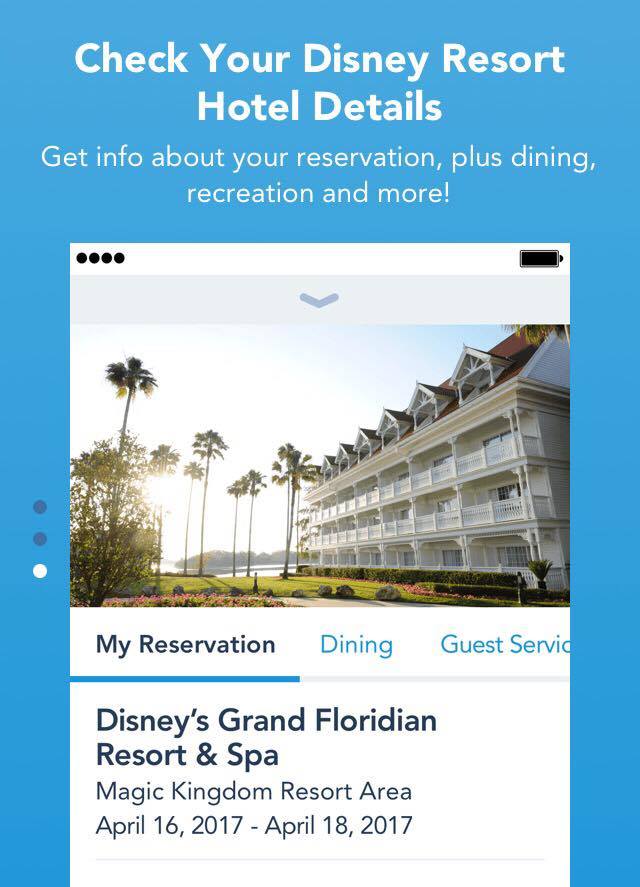The advertisement features a vibrant blue background adorned with bold white text at the top, proclaiming, "Check Your Disney Resort Hotel Details." Below this, in a smaller but still prominent font, it invites viewers to "Get info about your reservation, plus dining, recreation, and more."

At the center of the composition, a screenshot photograph of the Disney Grand Floridian Resort and Spa captures attention. This elegant image showcases the resort's grandeur with towering palm trees set against a pristine blue sky. The resort's iconic white, four-story building is prominently displayed, complete with ornate white balconies and graceful pillars.

Towards the bottom of the ad, a navigation bar features three tabs: "My Reservation," which is underlined in blue, suggesting it's the selected option; "Dining," also in blue; and "Guest Services." Furthermore, the text confirms the resort's full name and location: Disney Grand Floridian Resort and Spa, situated in the Magic Kingdom Resort area.

This advertisement effectively blends visual appeal with concise, informative text to entice viewers to check their Disney Resort Hotel details and explore the various amenities offered.